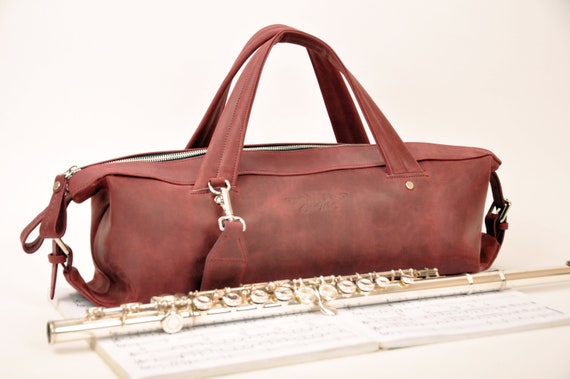This close-up photograph features an ensemble of musical elements set against a solid white background. At the forefront, there's an open book of sheet music lying flat. The pages, though slightly blurry, reveal scribbled musical notations. Horizontally positioned across the sheet music is an unassembled silver flute, showcasing its key mechanisms but sans the mouthpiece.

Behind the flute, a prominent brown leather bag sits snugly. The bag, likely a duffel or carrying case for the flute and sheet music, features two small handle straps on the top for easy lifting. It is adorned with multiple adjustable buckles on the sides and a zipper along the top edge. The bag's robust design suggests it's meant for secure and convenient transport of musical instruments and accessories.